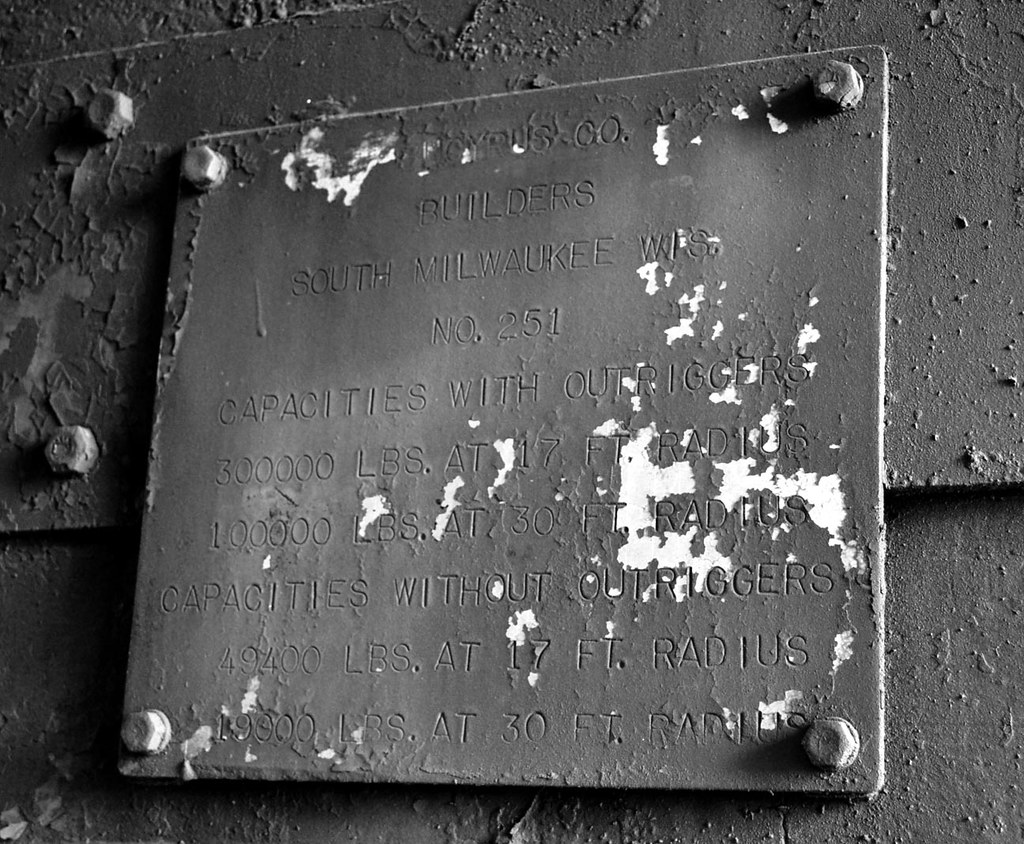In this black-and-white image, we see an old, weathered metal sign affixed to a similarly decrepit, possibly metallic wall using bolts in each corner. The sign is notably aged, with extensive chipping paint and signs of rust, though the grayscale of the image prevents any discernible coloration of the rust or paint degradation. The sign has engraved words, though some parts are partly illegible due to wear over time. The text on the sign reads "Eucharist Co. Builders, South Milwaukee WFS number 251." It lists weight capacities both with and without outriggers: "Capacities with outriggers - 300,000 pounds at 17-foot radius, 100,000 pounds at 30-foot radius; Capacities without outriggers - 49,400 pounds at 17-foot radius, 19,000 pounds at 30-foot radius." Despite the deteriorating conditions, the functional details remain notable on the sign, set against the backdrop of its multi-layered, scuffed metallic surroundings.